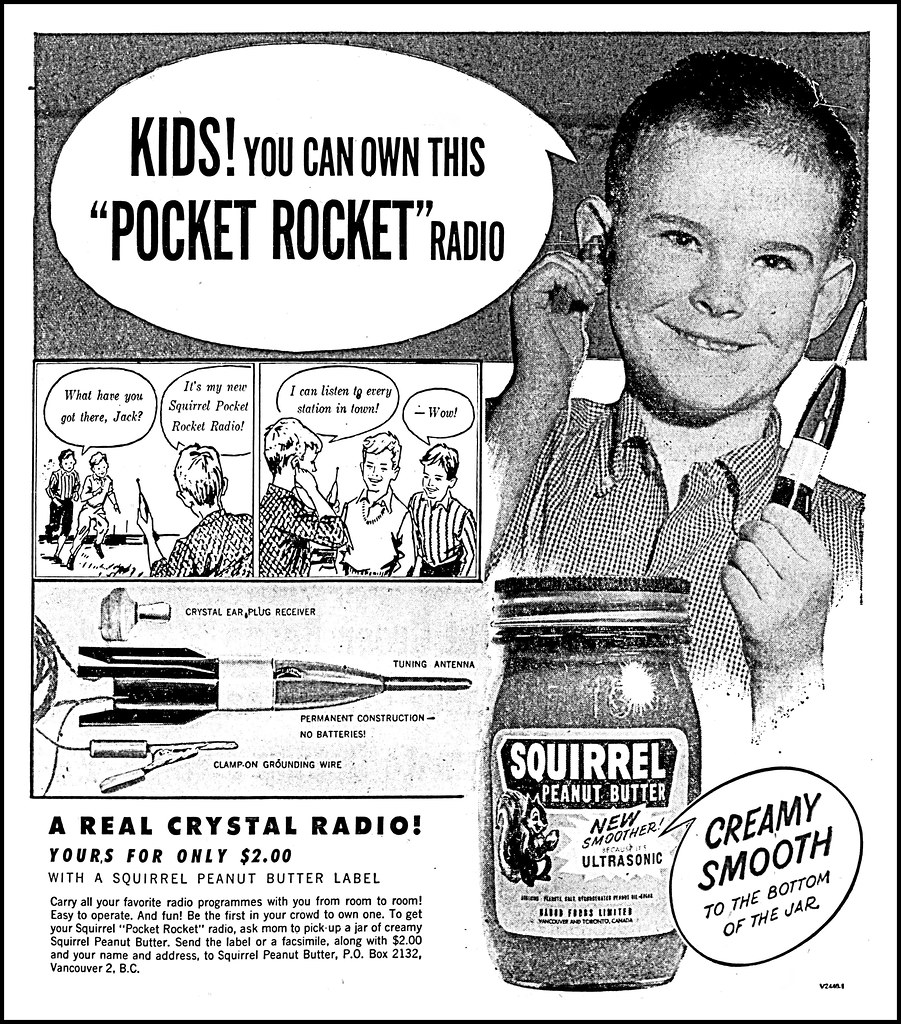This black and white image, evocative of a 1950s-era newspaper clipping or advertisement, showcases a young, approximately 10-year-old boy with a beaming smile, prominently holding a small black object resembling a pocket rocket radio. The boy is notably larger than the other elements in the image and stands towards the right side of the poster. In front of him, there is a jar of Squirrel Peanut Butter, emblazoned with a squirrel and the tagline, “Creamy smooth to the bottom of the jar.”

To the right of this jar, three smaller images are arranged vertically: two cartoon images at the top depict groups of people interacting, while the longer bottom image features a close-up of an arrow-like design with various labeled features. Adjacent to these images, a text block declares, “A real crystal radio. Yours for only two dollars.” A black shaded text box is positioned behind the boy’s head, perhaps indicating additional promotional text. Overall, the image is bordered in black and maintains a high-quality print for its era.